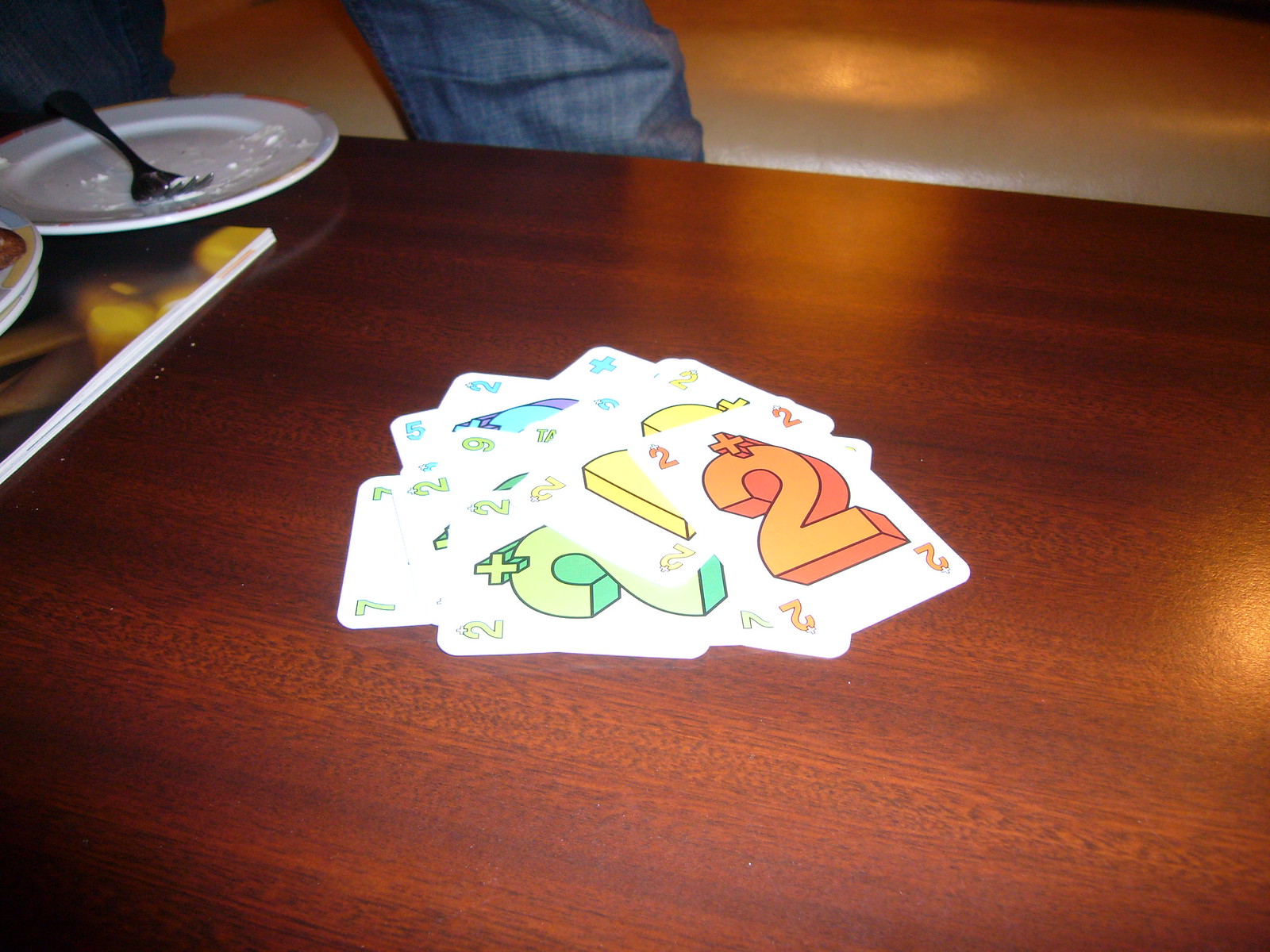A collection of white flashcards adorned with numbers is spread out on a richly stained, grainy wooden table. The surface is dark and appears to be of high quality, providing a striking contrast against the flashcards. Each card features a large, three-dimensional number in vibrant colors with a small, white plus sign above it. The most prominent card showcases an orange "2" in the center, surrounded by smaller orange twos in each corner, also marked with tiny white plus signs. 

Beneath the top card, a partially visible card displays a bright yellow number "2", with similar yellow twos in its corners. A green card with a number "2" peeks out from underneath, following the same design pattern. Other numbers, such as a green "9", a green "7", and a green "5", can be discerned within the shuffled stack of cards.

To the left, a white plate containing some crumbs and a dark-colored fork—likely silver—suggests a recently finished meal. The edge of another plate, possibly part of a stack, is just visible beside it. In the background, a pair of human legs clad in blue denim jeans and a light-colored floor can be seen, completing the scene.